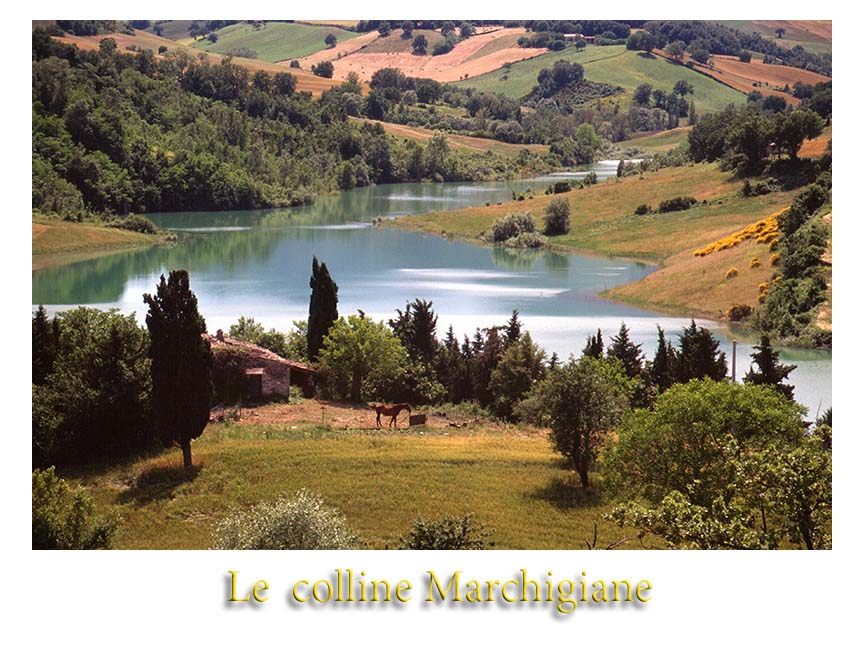The photograph captures a breathtaking outdoor landscape, primarily focusing on the environment and natural features rather than any single object. In the foreground, there is a small island with a few trees and a grassy area, where a horse stands near a small hut or building, and perhaps a box. This island is surrounded by a small body of water that resembles a pond or pooled section of a river. The water stretches towards the top right-hand side of the image, creating a serene focal point at the center.

On either side of the water, the land rises into rolling hills characterized by varied vegetation. Short trees and bushes populate these hills, with patches of brown and green grass interspersed. Notably, there are some yellow bushes present on the right side, adding a splash of color. Beyond the immediate foreground, the landscape continues with more hills and greenery, extending into the distance.

The sky above is clear, indicating a sunny, pleasant day. At the bottom of the image, the text "Les Collines Marchégiennes" is inscribed in yellow print, providing a title or description in a different language. The image's composition and vibrant colors of brown, green, blue, gray, and yellow capture the essence of a picturesque scene that might be shared on a website showcasing a specific area's natural beauty.